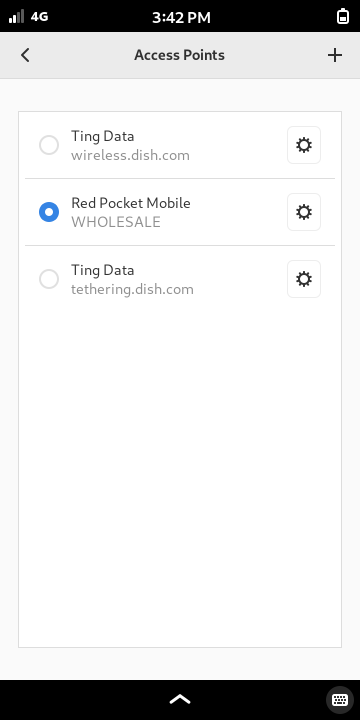A plain and simple screenshot of a mobile device screen is displayed. At the top, there's a black status bar with white icons and text. On the left of the bar, signal strength is shown alongside "4G." In the center, the time reads 3:42 p.m. On the right, a battery icon appears half-full. Below the status bar, a very pale blue navigation bar is visible. On the left of this bar, there's a back arrow, and on the right, a plus sign. Centered in this bar, "Access Points" is written in black lettering.

The main section of the screenshot shows three listed access points, each accompanied by a radio button and a gear icon on the right. The first access point is not selected and reads "Ting Data," with "wireless.dish.com" displayed underneath. The second access point is selected, indicated by a blue radio button, reading "Red Pocket Mobile," with "WHOLESALE" in all caps underneath. The third access point, also not selected, reads "Ting Data," with "tethering.dish.com" displayed underneath. The screenshot also shows a black footer bar at the very bottom with an upward-pointing arrow in the center.